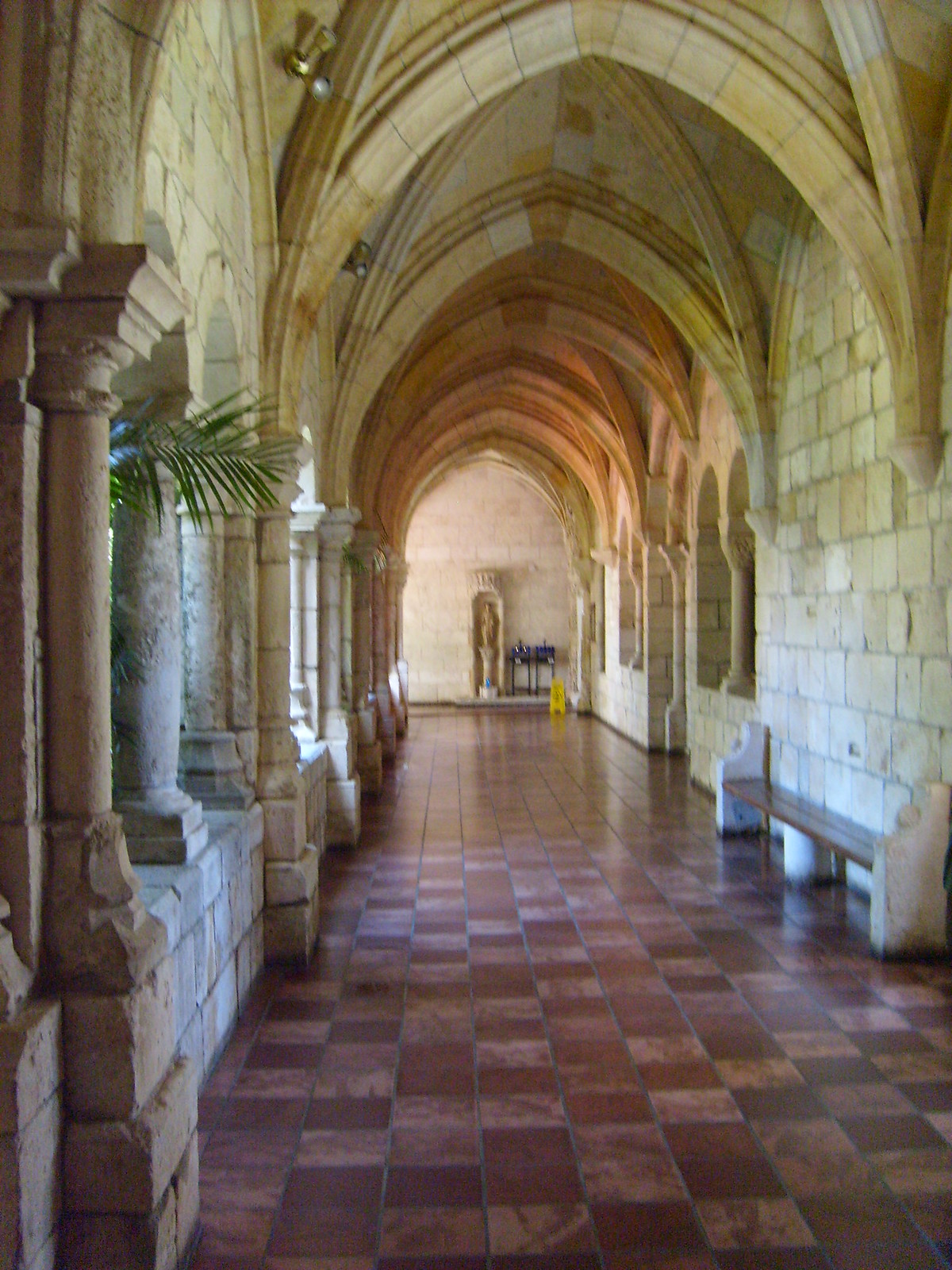The photograph captures a detailed view of an older, interior hallway in a church or cathedral-like building, characterized by its architectural features. The hallway, with high ceilings, is lined with white brick walls and dotted with sequences of white columns more prominent on the left side, creating an array of arches that span overhead. The floor is meticulously tiled in a checkered pattern of light and dark brown squares. A stark yellow caution sign is placed on the floor, drawing attention amidst the classic elements. A bench with a brown top is visible along the right side beneath the arches. In the distance, the hallway concludes at a wall adorned with what appears to be a piece of artwork or a statue. Additionally, a part of a green palm tree intrudes slightly into the space, adding a touch of nature. The composition of the image evokes a sense of historic and religious ambiance, amplified by the presence of a figurine against the opposite wall and the careful interplay of light and shadow throughout the scene.